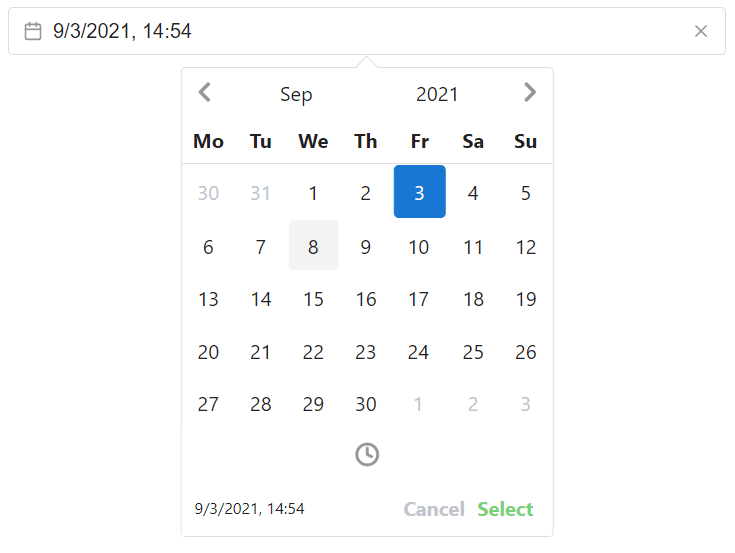The image depicts a detailed digital calendar interface. At the top, there's a rectangular section outlined in gray. Within this section, on the left-hand side, there is a small gray calendar icon. Adjacent to this icon, in black text, is the date and time, formatted as "9/3/2021, 14:54", indicating September 3rd, 2021, at 2:54 PM. On the right-hand side of this top section, there is a gray 'X' icon.

Below this section, there is a larger rectangle featuring navigation arrows on each side in gray, with a prominent "SEP 2021" (for September 2021) in the center. The days of the week are listed in bold black text as "MO" for Monday, "TU" for Tuesday, "WE" for Wednesday, "TH" for Thursday, "FR" for Friday, "SA" for Saturday, and "SU" for Sunday.

The calendar grid starts with numbers 30 and 31 in black from the previous month, with the date '3' highlighted within a blue box with white text for September 3rd. The dates continue sequentially through the month. The number '8' is highlighted with a gray box. The dates progress all the way to '30', after which the numbers turn light gray, indicating they belong to the next month.

At the bottom right corner, there's a small gray clock icon. In the bottom left corner of the image, the date and time are repeated in black text as "9/3/2021, 14:54". Next to it, there are options labeled "Cancel" in gray and "Select" in green.